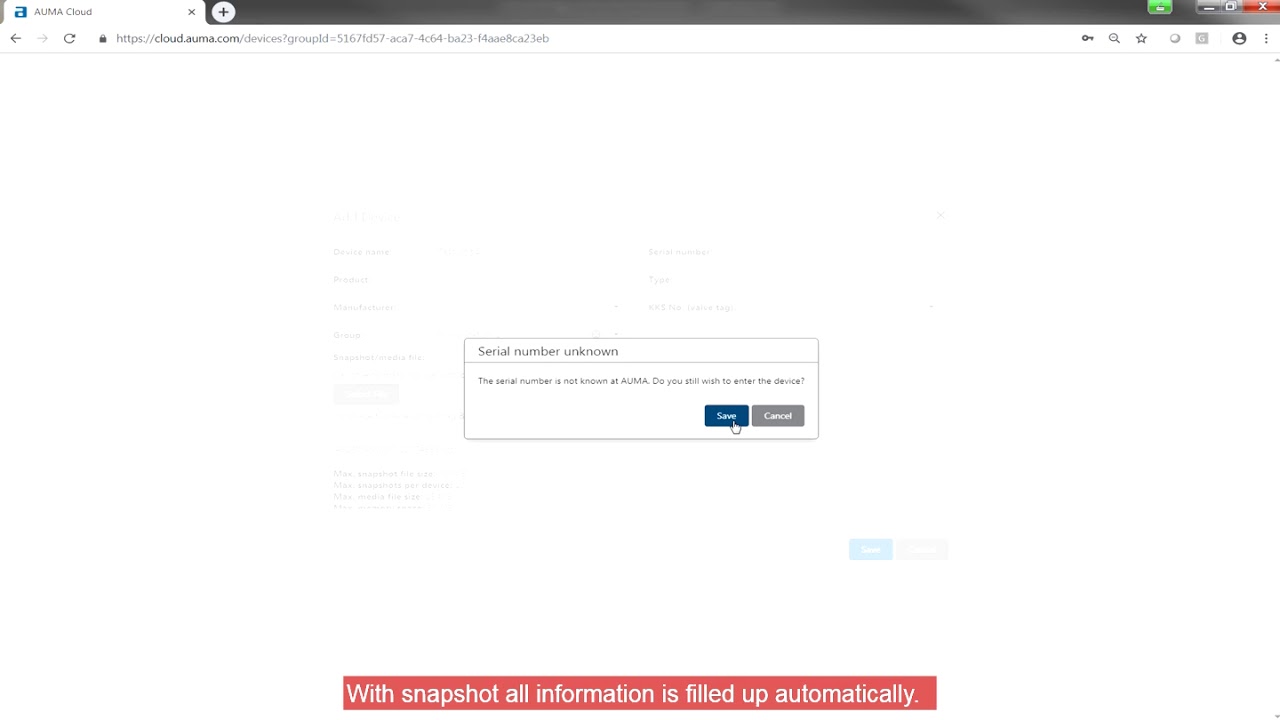The image depicts a partially loaded webpage with a white background. In the top left corner, there is a white tab indicating the page that is open, set against a black header background. The header includes white writing that presumably displays the website address, though it is illegible. To the right within the black header are three buttons: a green button, a gray button, and a red button featuring a white 'X'. Below this header, several icons are visible but indistinct, apart from a magnifying glass icon and an icon meant for a user profile image.

Dominating the middle section of the screen is a rectangular box labeled "Serial Number Unknown," accompanied by some inscrutable text. Below this text, there are two buttons: a blue button with white writing that likely reads "Submit" and a gray button with white writing that says "Cancel."

At the bottom of the page, there is a notable red bar with white writing that states, "With Snapshot, all information is filled up automatically." This red bar with its distinctive message is the most defining feature of the otherwise white-dominated page.